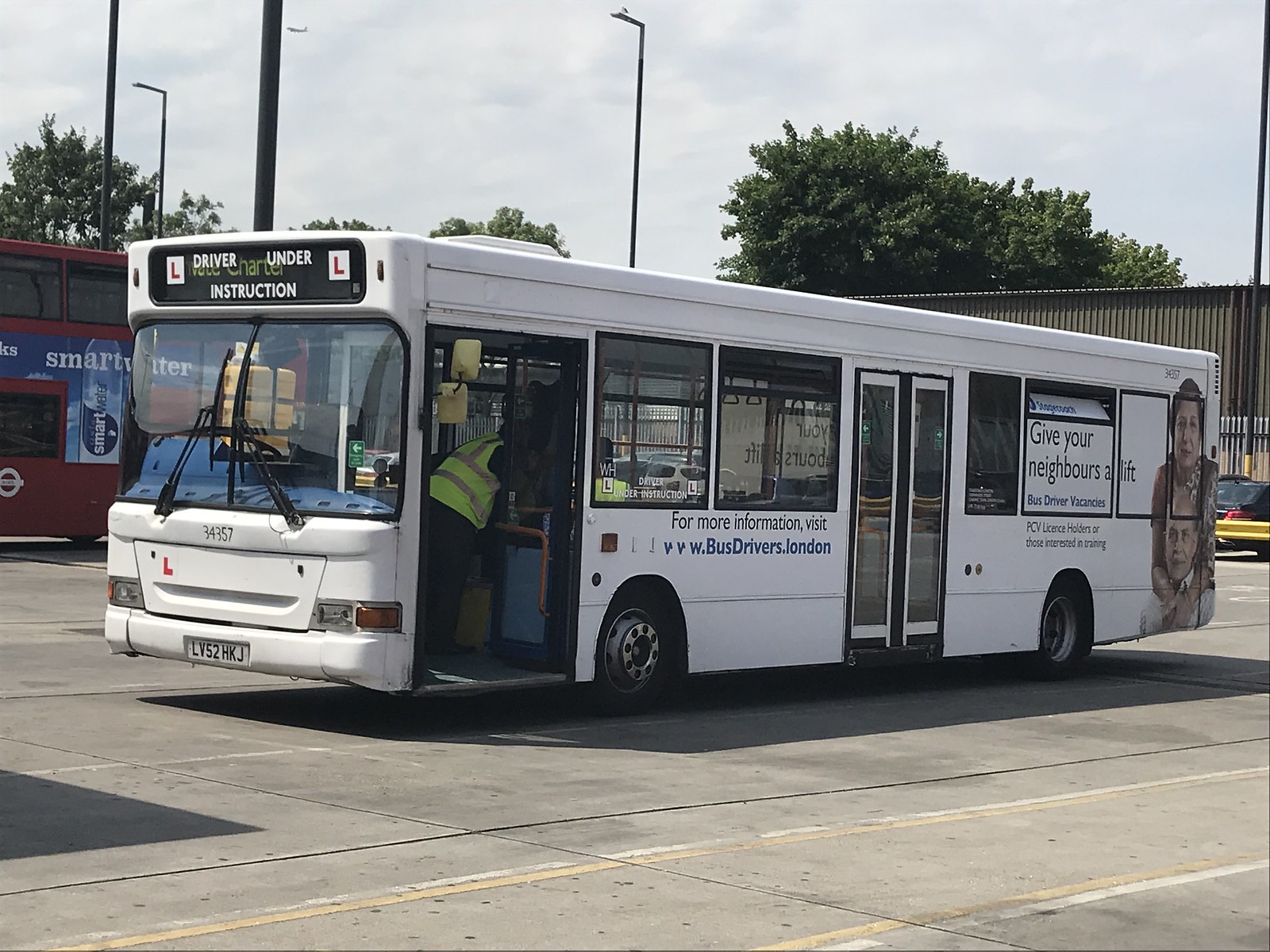This image depicts a detailed scene centered on a white single-decker bus parked on an asphalt road marked with yellow and white lane lines. The bus prominently occupies the center of the image and features several distinctive markings: at the front top, a sign reads "Driver Under Instruction" accompanied by two red L plates on either side. Below the windscreen, the bus has a black number "34357" and a license plate "LV52HKJ" on a white background. The front doors are open, and a person wearing a high-visibility vest stands in the doorway. 

Along the side of the bus, text reads, "For more information, visit www.BusDrivers.London," and towards the rear, overlaid on a window, another message says, "Give your neighbors a lift. Bus driver vacancies, stagecoach." The back of the bus features an image or sticker of an elderly couple. The scene is set outdoors, in the middle of the day, potentially at a bus depot, as suggested by the presence of another red double-decker bus and various objects in the background, including a black car, trees, poles with light posts, and a building. The backdrop displays a sky filled with clouds and a blue background. Additional details include a smart water bottle logo on a side element and some random text suggesting commercial markings, like "Nissan." The overall color palette includes varying shades of gray, white, yellow, blue, black, green, brown, and red.